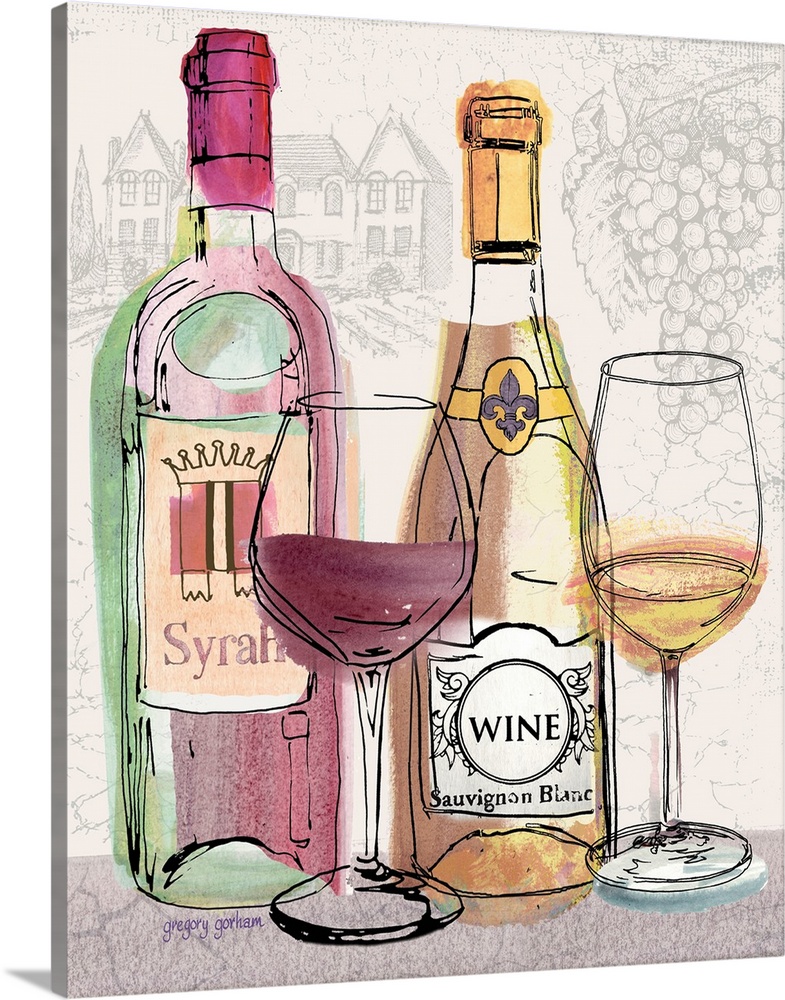The image is a vertically aligned rectangular painting on what appears to be a canvas or possibly wood, slightly tilted to reveal a solid gray left edge about an inch thick. This artwork, likely something you'd hang on the wall, features a mix of sketched and colored elements.

In the background, sketched in pencil, there's a large multi-story house in the upper left corner, possibly indicative of a wine vineyard, and a bunch of grapes in the upper right corner. The sketches lend a classic, unfinished charm to the setting.

At the forefront, vibrant in color, the painting showcases two bottles of wine and two glasses. On the left, the first bottle stands tall with a label reading "Syrah" in pink, adorned with an image of a crown and a square design in pink and green. It has a dark pink cap. In front of this bottle, a wine glass contains a purplish-pink liquid, matching the wine from the Syrah bottle.

The second bottle, positioned centrally, features a predominantly gold label with "Sauvignon Blanc" written in black text. It has a gold cap and contains a golden-brown liquid. A wine glass to its right is quarter-filled with this light amber liquid.

The bottom left of the painting has the artist's signature, "Gregory Gorham," in small purple text. Overall, the composition brings together elements of both realistic color and pencil sketching, depicting a wine-themed scene with meticulous detail.